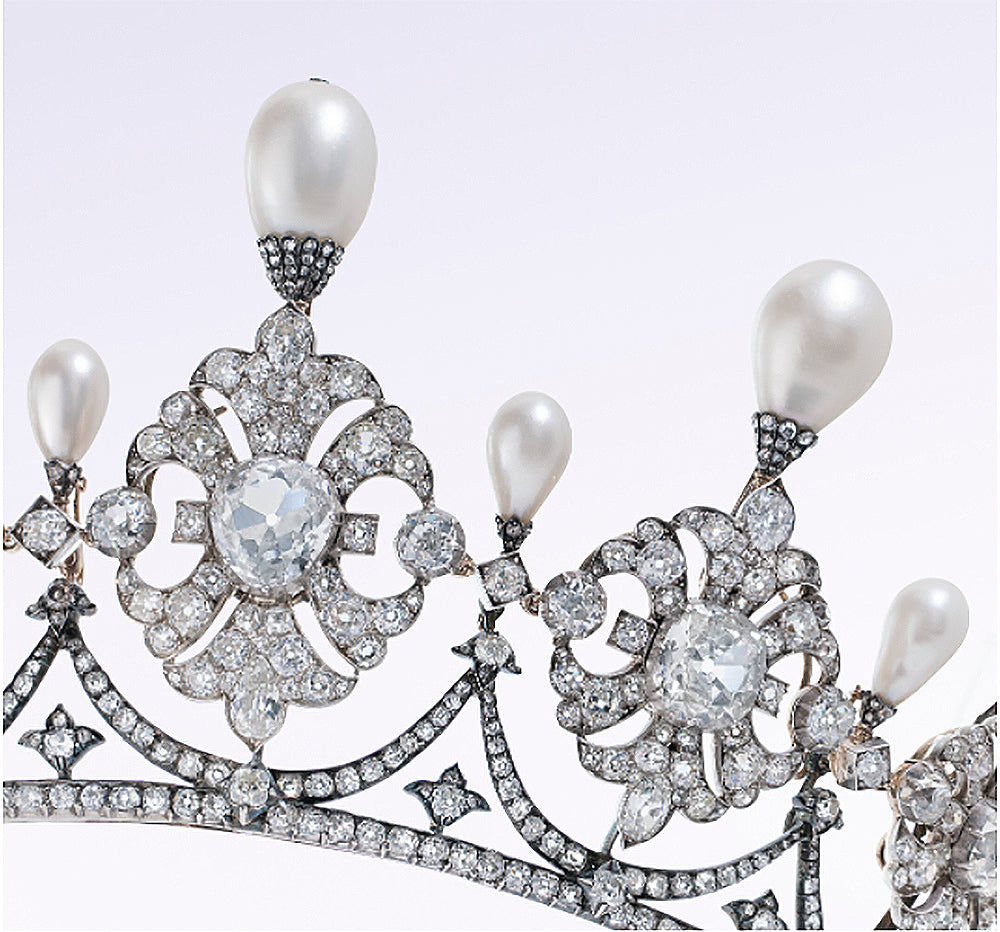The image is a close-up photograph of a crown or tiara with a solid white background. The piece is lavishly adorned with various shiny stones, primarily diamonds of multiple shapes and sizes, including large round and square cuts. Each tip of the crown is accented with oval, egg-shaped pearl-like figures, adding to its intricate design. The design incorporates interconnected fleur-de-lis symbols beneath the pearls, connected by diamond-shaped elements featuring a smaller diamond within each and topped with shorter pearls. Semi-circle elements support these designs, creating a unified and elaborate pattern. The crown's lower band secures the overall structure, making it an opulent piece that appears to be almost entirely covered in diamonds and pearls, suggestive of royal ownership and immense value.